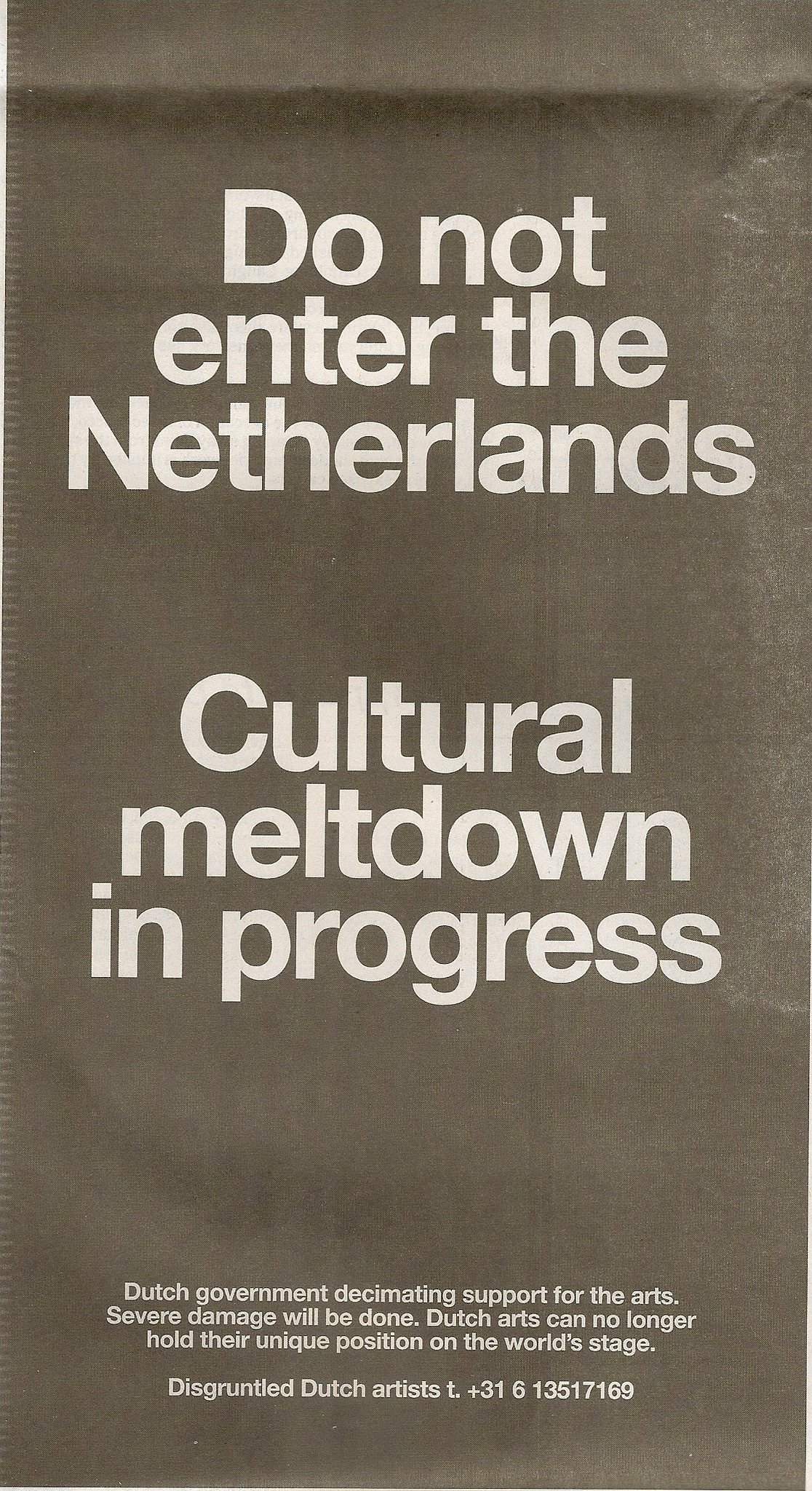Here is a cleaned-up and combined caption based on the given descriptions:

The image is a vertical rectangular ad printed on an old, fabric-like textured material with a washed-out grey-black background. At the top, large white bold letters state, "DO NOT ENTER THE NETHERLANDS." Below this, it continues with, "CULTURAL MELTDOWN IN PROGRESS." Towards the bottom, in smaller white font, it reads, "Dutch government decimating support for the arts. Severe damage will be done. Dutch arts can no longer hold their unique position on the world stage." The message concludes with, "Disgruntled Dutch artist," followed by the contact detail, "T. +31 6 13517169." Additionally, there is an imprint on the top right of the image.